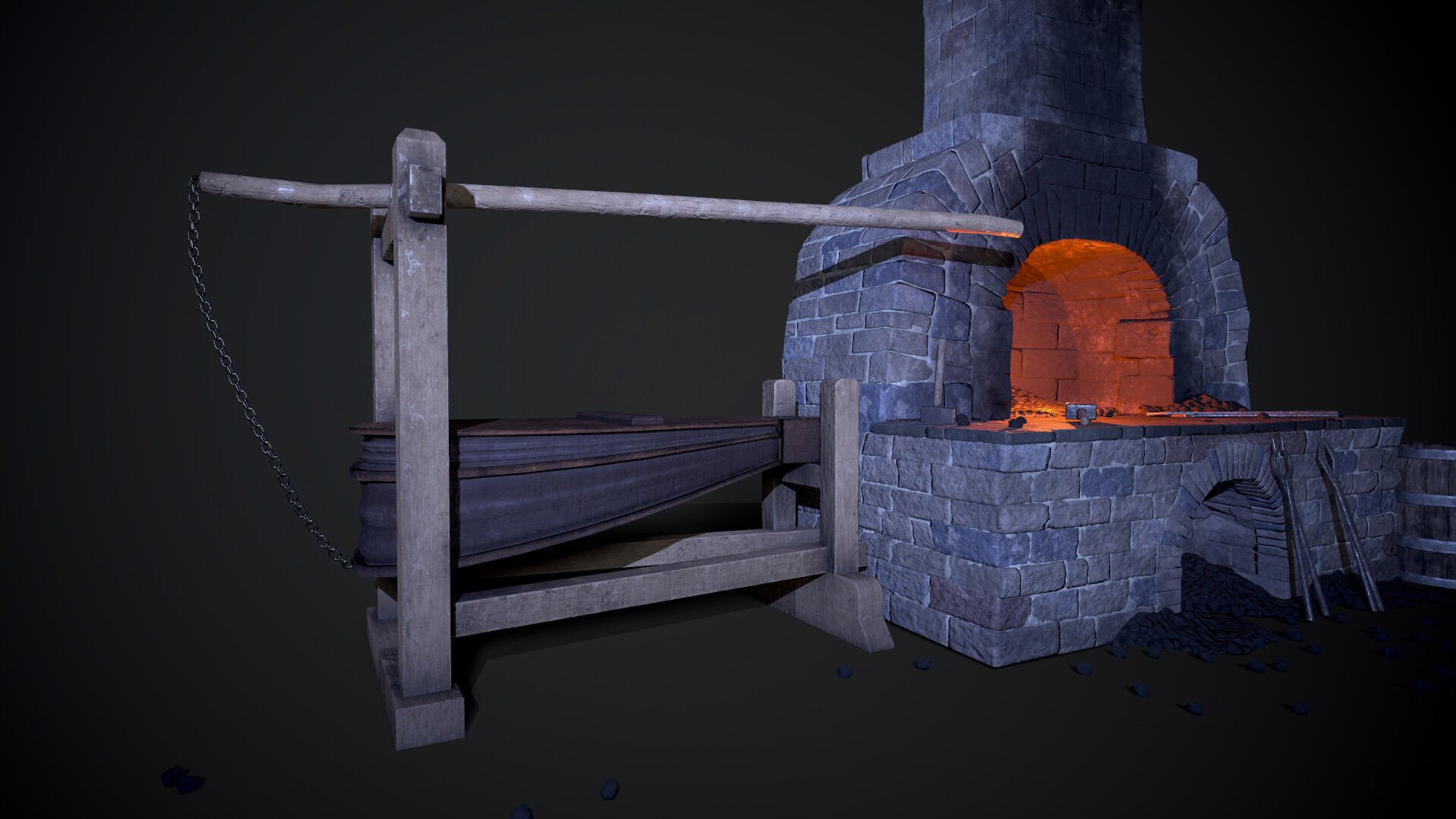The image depicts a large, old-style brick fireplace with a distinct arched opening for the fire materials and a smaller arch at the bottom for cleaning out the area. It's constructed from gray and tan stone, with a chimney column extending upward from the main arch. The background of the scene is quite dark, with the fireplace glowing orange from an inferred fire, casting a warm light. On the wooden structure to the left of the fireplace, there's an apparatus resembling a bellows, designed to fan the fire by inflating and deflating an accordion-like airbag. This bellows mechanism is activated by a long wooden pole connected to a chain. The fireplace stands on a brown floor, and several fire-tending tools lean against or hang from the structure, adding to the authentic rustic ambiance of the scene.